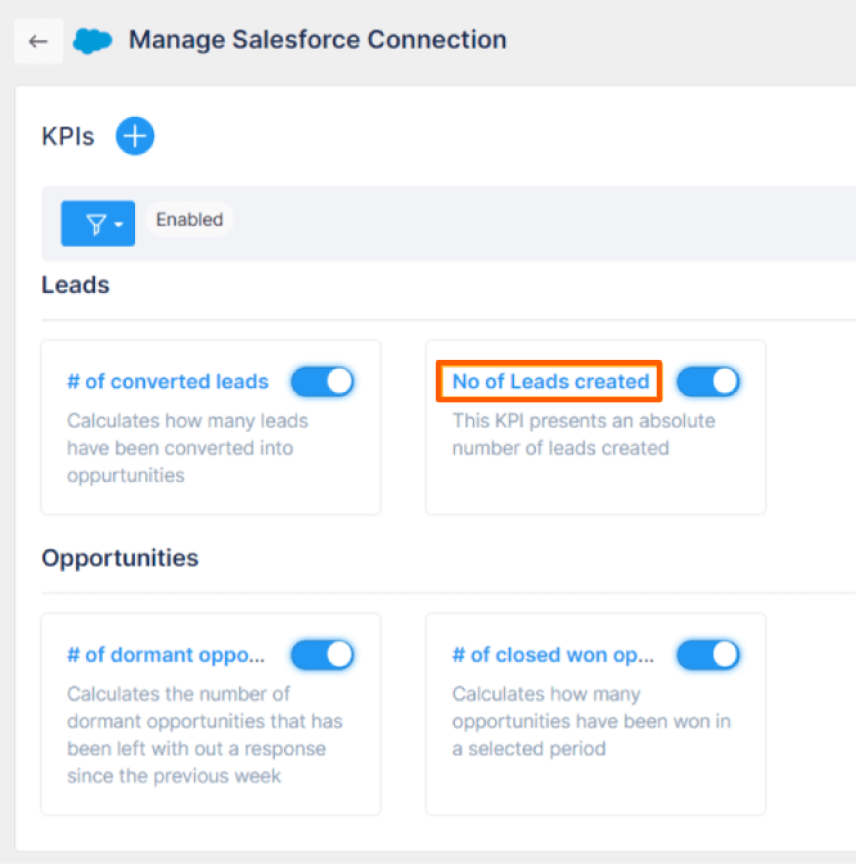**Webpage Screenshot of Salesforce Management Interface**

The image captures a webpage dedicated to managing Salesforce connections. The top navigation bar features a back arrow icon and a cloud icon, with the header text reading "Manage Salesforce Connection."

**KPIs Section:**
- A blue circle with a white plus sign is present, accompanied by a light indicator with a blue background labeled "Enabled."

**Leads Section:**
- The first box is titled "Number of Converted Leads." It contains a blue button indicating it is turned on. Below it, gray text reads, "Calculates how many leads have been converted into opportunities."
- The second box is titled "No Leads Certified," highlighted with an orange text box. The description states, "This KPI presents an absolute number of leads created."

**Opportunities Section:**
- The first box is titled "Number of Dormant Opportunities." It includes a blue box with text explaining, "Calculates the number of dormant opportunities that have been left without a response since the previous week."
- The last box is titled "Number of Closed Won." Partial text indicates "OP..." and it also features a blue button indicator. Gray text below states, "Calculates how many opportunities have been won in a selected period."

The overall layout features a white background with black and gray text, enhanced by blue buttons and indicators for interactive elements.